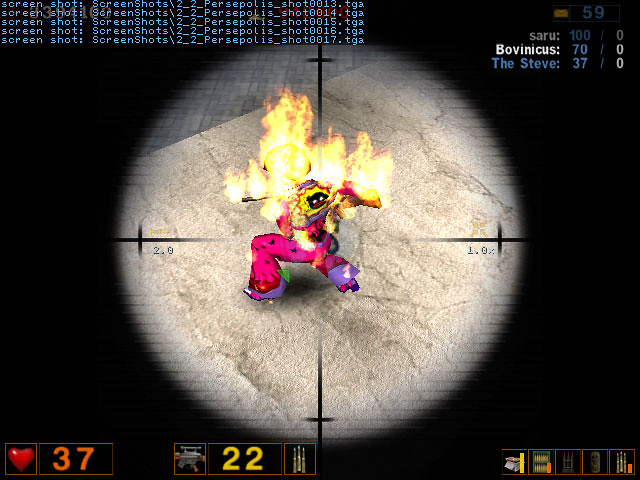This detailed caption accompanies a screenshot from a video game, emphasizing various on-screen elements and features present in the image:

---

The screenshot, marked as "screenshot\screenshots\2_2_per_SEPOLIS_SHOTO_0013.TGA" in the upper left corner, is one in a series of similar images, each with slight variations in their file names. On the right-hand side of the screen, the interface displays the text "SARU 100 BOVINICUS 70/0" and below it "Steve: 37/0," possibly indicating player statistics or character information.

Dominating the center of the image is a prominent gray circle set against a black background. Within this circle, a figure resembling a clown is depicted. The clown wears a yellow mask featuring black eyes, and its attire includes a striking pink suit with purple accents. This clown appears to be engaging in a performance, possibly twirling batons that are aflame, adding a dynamic and intense element to the scene.

At the very bottom left of the screen, additional visual and numerical details are present. A heart icon is displayed next to the number 37, followed by an icon of an image or item labeled 22, and further accompanied by other small, undecipherable images, contributing to the complex and intricate visual layout of the game interface.